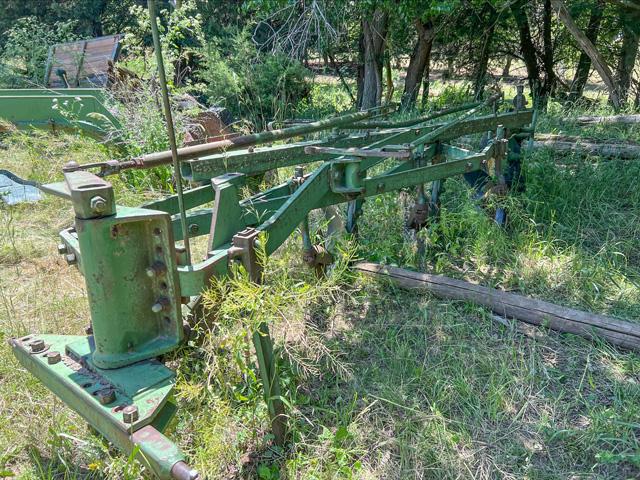The photograph captures an old John Deere bottom plow with faded green paint, abandoned in an overgrown, unkempt field or backyard. The scene is dominated by greenery, with tall weeds growing up through and around the plow, alongside other disused farming equipment. This area, filled with trees, bushes, and patches of sunlight, reveals signs of previous human activity, including felled trees and remnants of what appear to be wooden posts from a fallen gate. The overall impression is one of nature reclaiming space, enveloping the neglected machinery that once played a crucial role in farming.